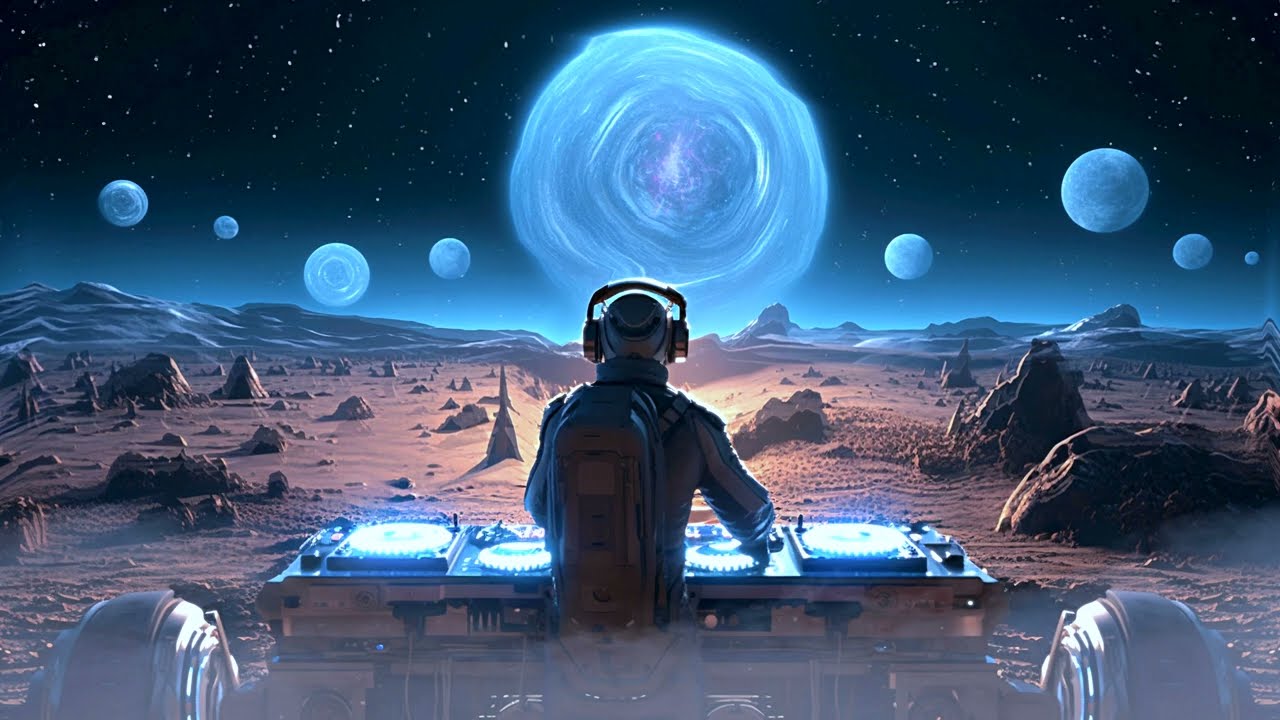In this detailed, computer-generated 3D rendering, a humanoid figure, depicted as a DJ, stands on a barren, rocky alien planet. The scene is viewed from behind the DJ, who is equipped with a backpack, wearing a long-sleeved shirt reminiscent of a motorcycle jacket, headphones, and a hat. The DJ is stationed in front of a futuristic, sci-fi DJ turntable apparatus, which intriguingly features wheels on either side, perhaps giving it the appearance of a rover. 

The Martian-like landscape is characterized by sharp rock formations, tall spires, scattered boulders, and rolling hills stretching toward the horizon. The sky is a mosaic of interstellar wonders: a vast, starry night dotted with numerous moons, including one particularly large and swirly celestial body. Dominating the center of the scene is an enigmatic blue and purple portal or wormhole, exuding a mysterious hue that casts a bluish tint over the distant terrain. This cosmic vista combines the dark void of space with the captivating celestial phenomena, painting an awe-inspiring backdrop for the lone DJ immersed in his otherworldly performance.